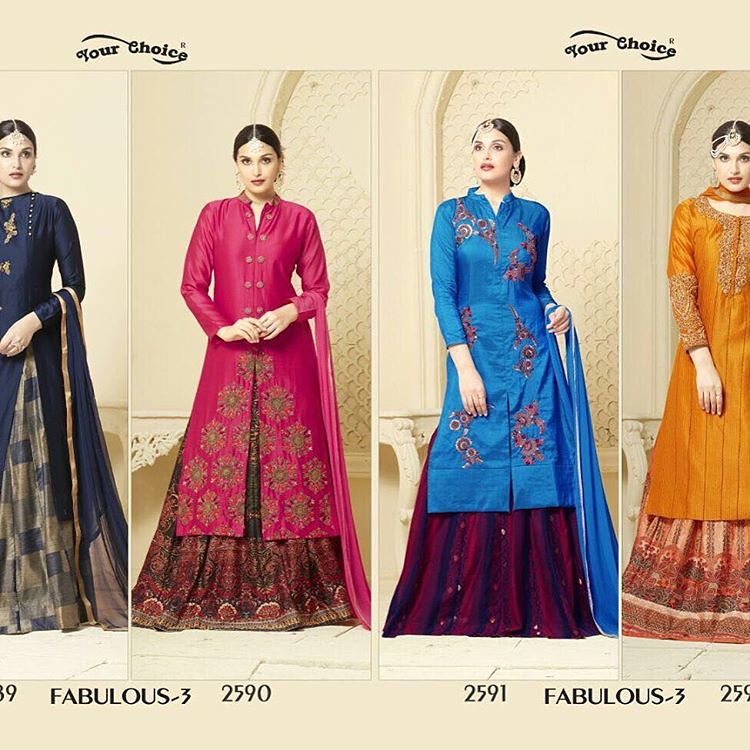This square advertisement showcases a model in four traditional Indian dresses against a tan background, with the text "Your Choice" prominently displayed at the top. The model appears partially on the far left and right but is fully visible in the middle two panels. At the bottom, the image is marked with "Fabulous-3" and price tags of $25.90 and $25.91.

The model consistently wears her straight brown hair slicked back with a middle part and large hoop earrings. Starting from the left, she dons a navy blue dress with a long train. In the second panel from the left, she wears a dark pink dress adorned with gold patterns at the hem. The third panel features her in a striking bright blue dress with a burgundy-colored bottom, while the far-right panel showcases her in a gold-patterned dress with a multicolored floral bottom.

The advertisement, brimming with vibrant colors and intricate patterns, beautifully presents these traditional Indian garbs, each priced just over $25.